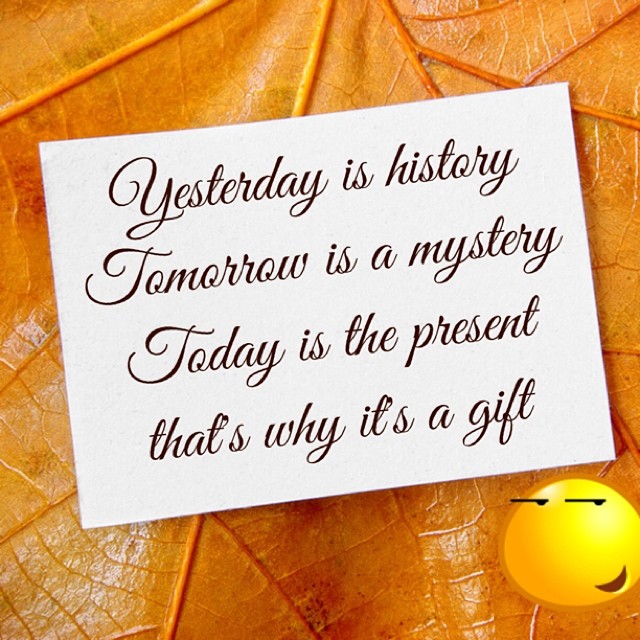The image displays a close-up, textured background of a shiny, deep orange-yellow leaf with prominent veins. Atop the leaf is a slightly rotated, off-white card featuring dark brown cursive text. The inspirational quote on the card reads: "Yesterday is history, tomorrow is a mystery, today is the present, that's why it's a gift." In the bottom right corner, a modern yellow emoji with slanted eyes and a sly, sideways smile adds a touch of whimsical wisdom to the scene, resembling a motivational meme one might share on social media.